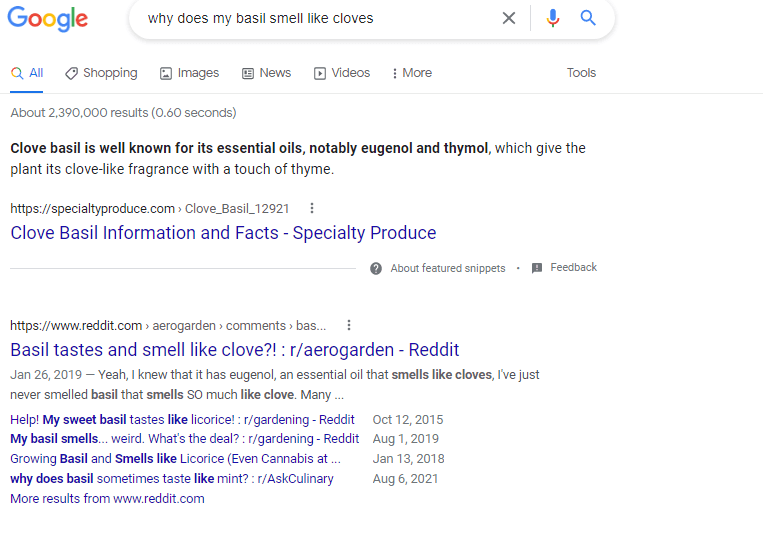The image captures a Google search query page where someone has typed in "why does my basil smell like cloves?" At the top, the iconic Google logo appears in colorful letters. Below the search bar, there are navigational tabs for different categories including All, Shopping, Images, News, Videos, More, and Tools.

The search results highlight the primary reason: the presence of essential oils such as eugenol and thymol in clove basil, which contribute to its clove-like fragrance with a hint of thyme. Below this explanation, various website links are listed, including a Reddit discussion from 2019 where a user confirms that eugenol is responsible for the clove-like smell in basil, expressing their surprise at how strongly their basil smells like cloves. Additionally, another query is visible where someone is concerned about their sweet basil tasting like licorice, indicating a variety of user-generated questions and answers related to basil's scent and flavor.